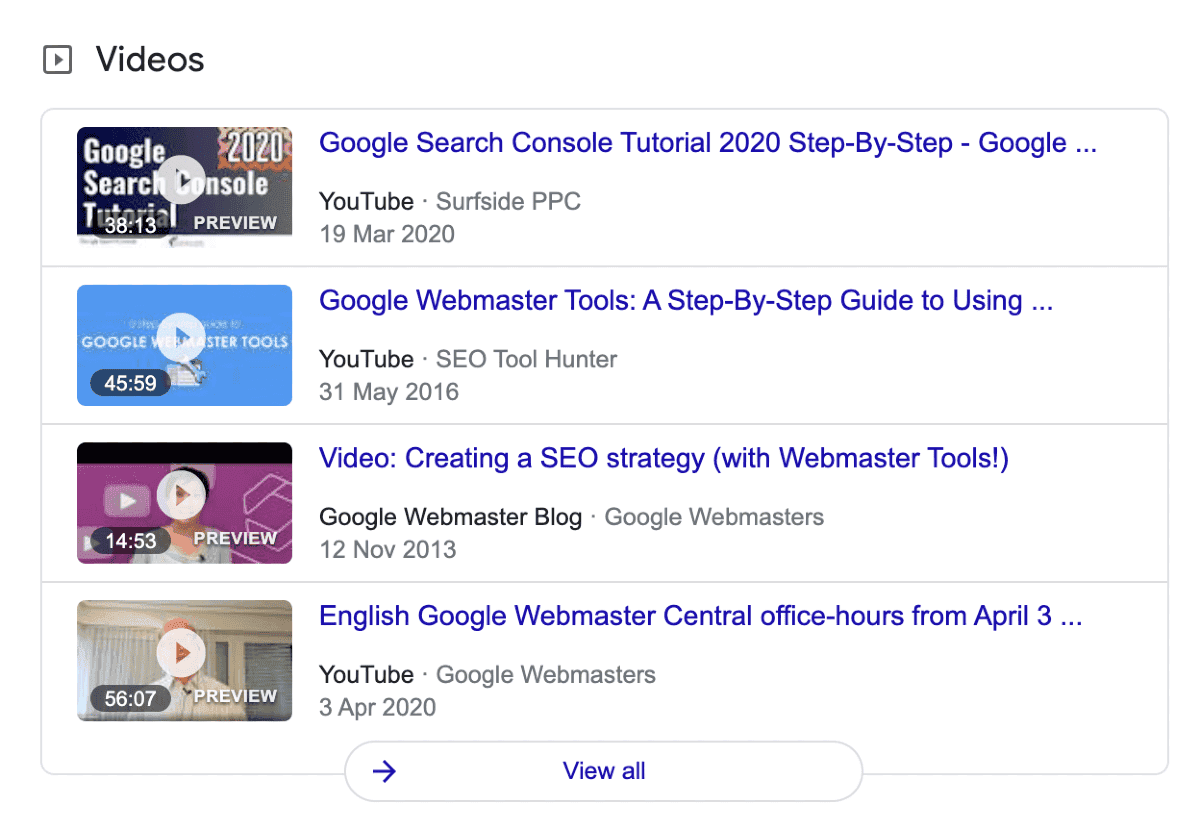A screen capture displays a Google search results page, specifically showcasing the "Videos" subsection. This section appears to have been cropped from the main search results page, indicated by a "View All" button at the bottom. The "Videos" subsection prominently lists four video tutorials focused on Google-related topics: 

1. "Google Search Console Tutorial"
2. "Google Webmaster Tools"
3. "Creating an SEO Strategy"
4. "English Google Webmaster Central"

The duration of these videos ranges from approximately 15 minutes to 56 minutes. The interface follows Google's typical design, featuring a clean white background and blue highlights synonymous with the Google brand. The presence of the "View All" button suggests this is part of a broader search results page rather than a dedicated video search.